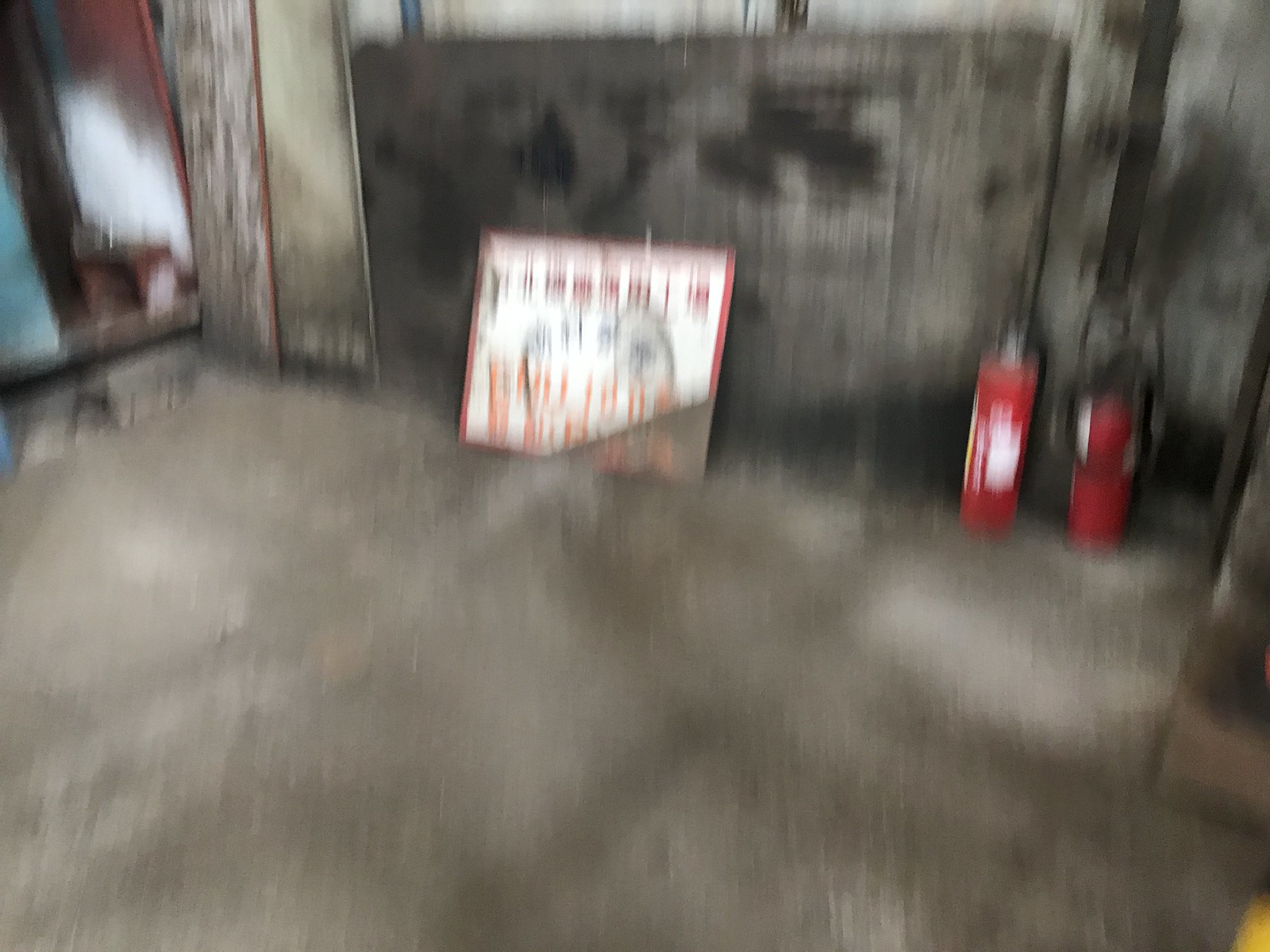The image depicts a very blurry scene in what appears to be an old, empty warehouse or barn with a concrete floor. Against the right side of a burned wooden wall are two tall, red fire extinguishers. The central focus of the picture is a billboard with predominantly white background and red Chinese writing, accompanied by larger orange lettering toward the bottom. Light seems to be filtering into the space, indicating it's daytime. On the left side of the image, several tall wooden boards are leaned against the wall, one of which is grayish, and another appears to have black lines. The lack of clarity makes precise description difficult, but these elements provide a general sense of the contents and setting of the image.